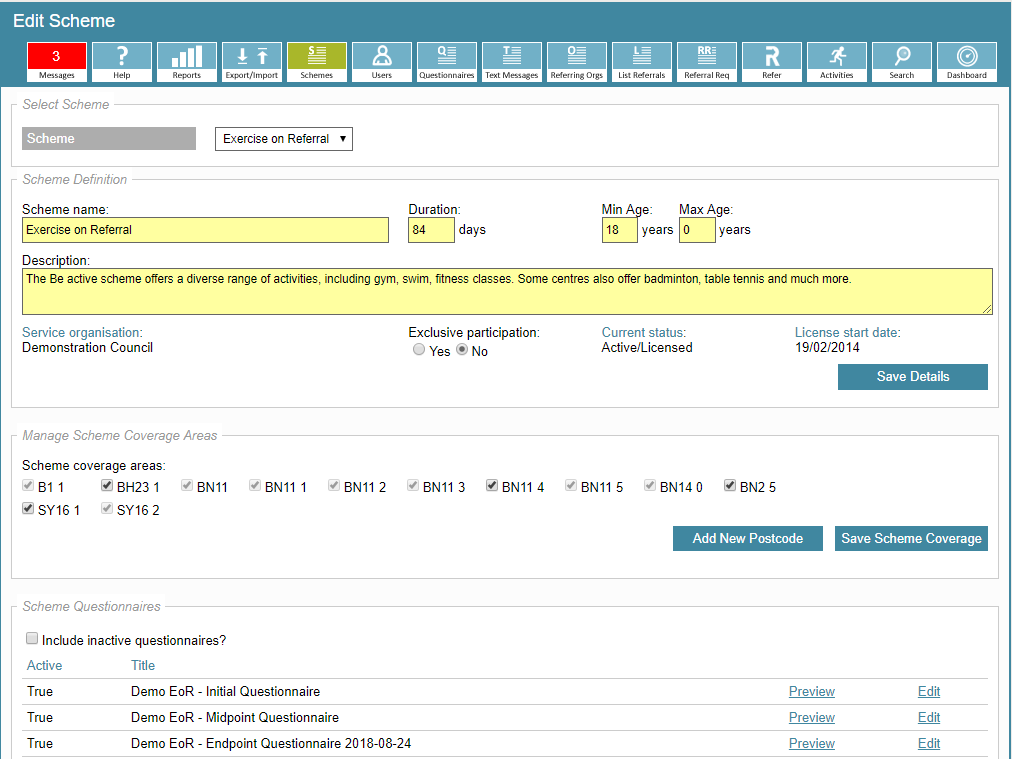**Detailed Image Caption:**

The image showcases a comprehensive management interface for a scheme, structured as a detailed spreadsheet. At the top of the screen, there is a toolbar featuring several buttons, namely: "Edit Scheme," "Messages" (with a notification badge displaying the number 3), and a "Help" button. These buttons are aligned horizontally alongside tabs labeled "Reports," "Export/Import," "Schemes," "Users," "Questionnaires," "Text Messages," "Referring Orgs," "List Referrals," "Referral Reg," "Refer," "Activities," "Search," and "Dashboard."

Beneath this toolbar, the section titled "Select Scheme" contains a drop-down menu in a gray box, labeled "Scheme," with "Exercise on Referral" already selected. The "Scheme Definition" further details the scheme name as "Exercise on Referral," with a duration of 84 days. The scheme specifies a minimum age of 18 and no maximum age (indicated by 0). Its description states: "The 'Be Active' scheme offers a diverse range of activities including gym, swimming, fitness classes, and some centers also offer badminton, table tennis, and much more." 

The "Service Organization" is listed as "Demonstration Council," and the "Exclusive Participation" option is set to "No." The "Current Status" reads "Active / Licensed" with a license start date of February 19, 2014. Additionally, there is a "Save Details" button to save the scheme information provided.

Further down, the "Manage Scheme Coverage Areas" section lists specific postcodes, which include: B1, BH23, BN11 (repeated multiple times), BN2, and SY16 (also repeated). Each of these coverage areas is marked with a checkbox. Below this, buttons for "Add New Postcode" and "Save Scheme Coverage" are available.

Lastly, the "Scheme Questionnaire" section offers options to "Include Inactive Questionnaires," along with buttons for activating questionnaires. Three specific questionnaires are listed: "Demo EOR Initial Questionnaire," "Demo EOR Midpoint Questionnaire," and "Demo EOR Endpoint Questionnaire." Each of these options can be previewed or edited.

This detailed interface aims to provide a highly organized and user-friendly means to manage various aspects of the "Exercise on Referral" scheme efficiently.